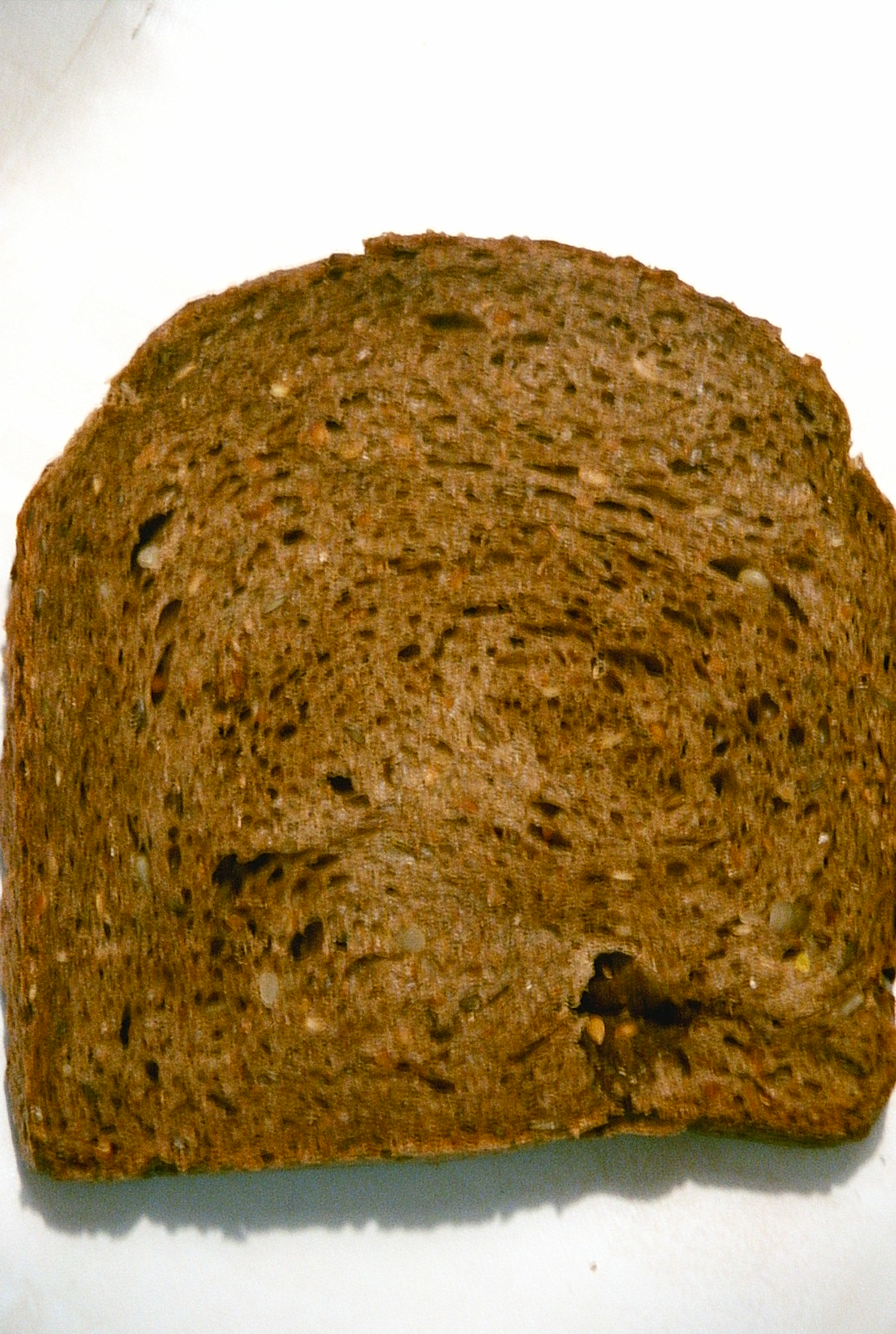This image showcases a slice of bread that, upon closer examination, appears to be banana bread. The bread is situated in the center of the photograph, which is taken from above, showing it laid on a white surface that might be a table or a plate. The slice is rectangular with a rounded top and a dark brown color, implying it might be toasted or slightly old. There are small seeds or specks visible throughout the bread, suggesting it could be a whole wheat variant. The lower right corner of the slice has a noticeable indentation and darker hue. The bread casts a slight shadow, hinting at its thinness. There is also some discoloration with a purplish hue in the upper left corner of the surface it rests on. Despite its plain and dry appearance, it looks delicious and inviting, evoking a sense that it would be enjoyable to eat.